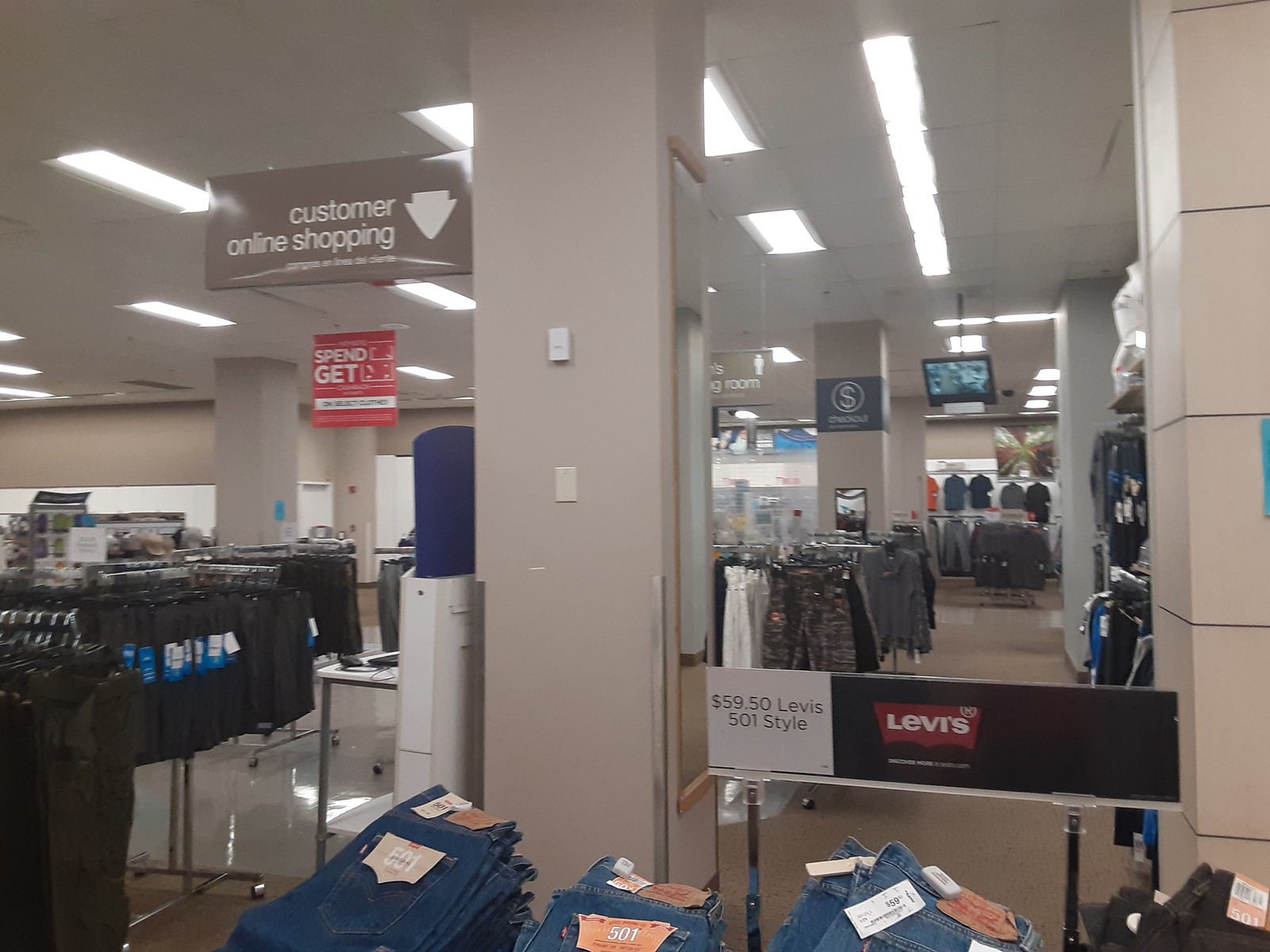This image captures the interior of a department store, characterized by its off-white walls, floor, and pillars. In the foreground, a table displays four stacks of Levi's jeans—three in traditional denim blue and one in gray. Behind the table, a prominent sign showcases the Levi's logo in red and white letters against a black background alongside a white area that reads "$59.50 Levi's 501 Style." This display is flanked by two beige columns, one made of bricks and the other plain with tan plates. Fluorescent lights illuminate the space, and several clothing racks populate the area with shirts, pants, and denim skirts. In the background, another room with shirts hanging from a white structure against a beige wall is visible. Additional signage includes a brown sign with white letters reading "Customer Online Shopping" and a video screen potentially used for security purposes. The scene is indicative of a typical department store setup, possibly resembling a Kohl's.